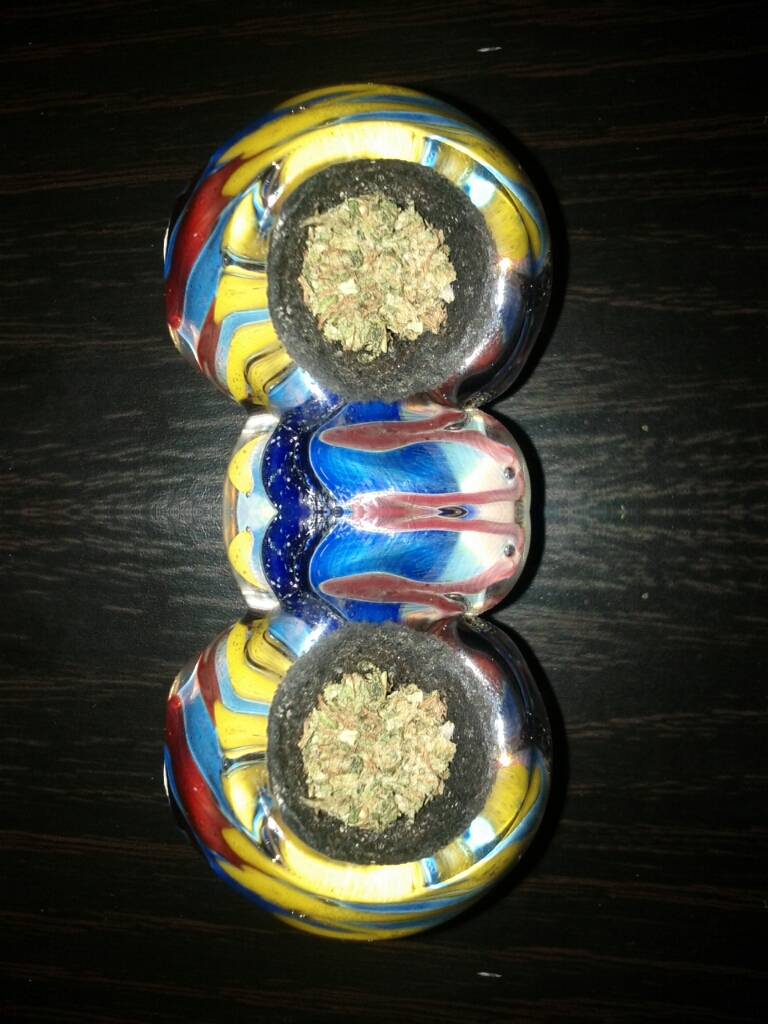This is an overhead photograph of a hand-blown glass pipe, intricately designed to resemble an elongated figure eight. The pipe features two symmetrical bowl sections at the top and bottom, connected by a narrower middle support structure. The vibrant, multicolored glass exhibits a liquid-like quality, swirling with hues of yellow, blue, and red, while the middle section is a lighter red with subtle blue streaks interlacing with darker shades. Both bowl sections contain flowered cannabis, and there is visible black residue indicating prior use. The photograph, taken on a black and dark brown wooden table with a horizontal grain, is harshly lit, highlighting the speckled gray color of the bowls and the intricate detailing of the glass artwork.